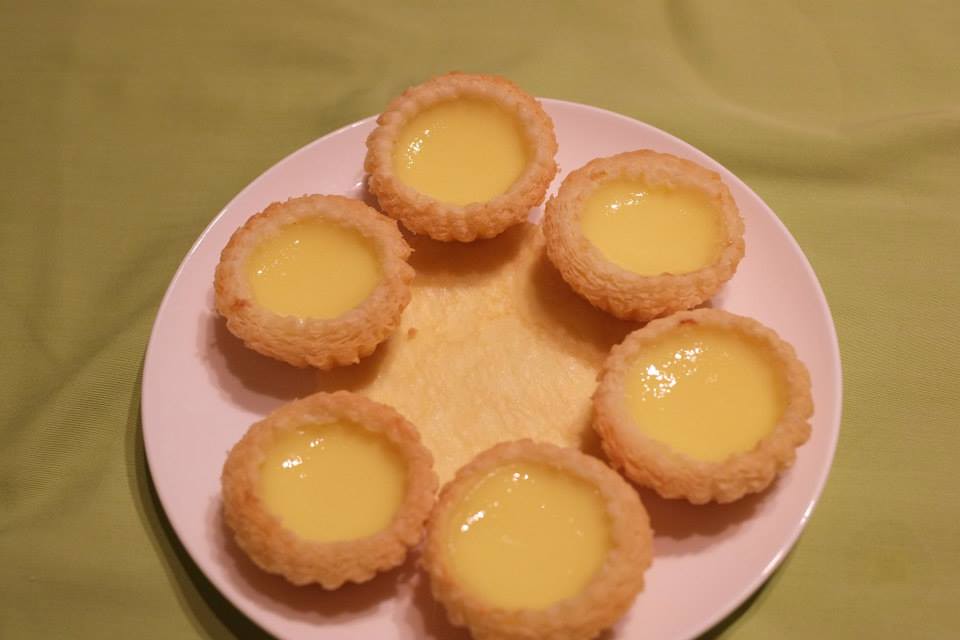The photograph features a pink plate set against a light greenish fabric background that exhibits subtle wrinkles, with a shadow cast by the plate on the lower portion of the image. Centrally arranged on the pink plate are six small, circular desserts, forming a precise ring. These desserts appear to be delicately crafted from a pie crust-like base, showcasing a light brown, slightly crispy exterior. Inside each dessert, there's a glossy, slightly runny yellow custard that catches the light, indicating a rich, creamy texture. At the very center of the plate lies a small, off-white circular piece of paper, possibly a napkin, adding a refined touch to the presentation.